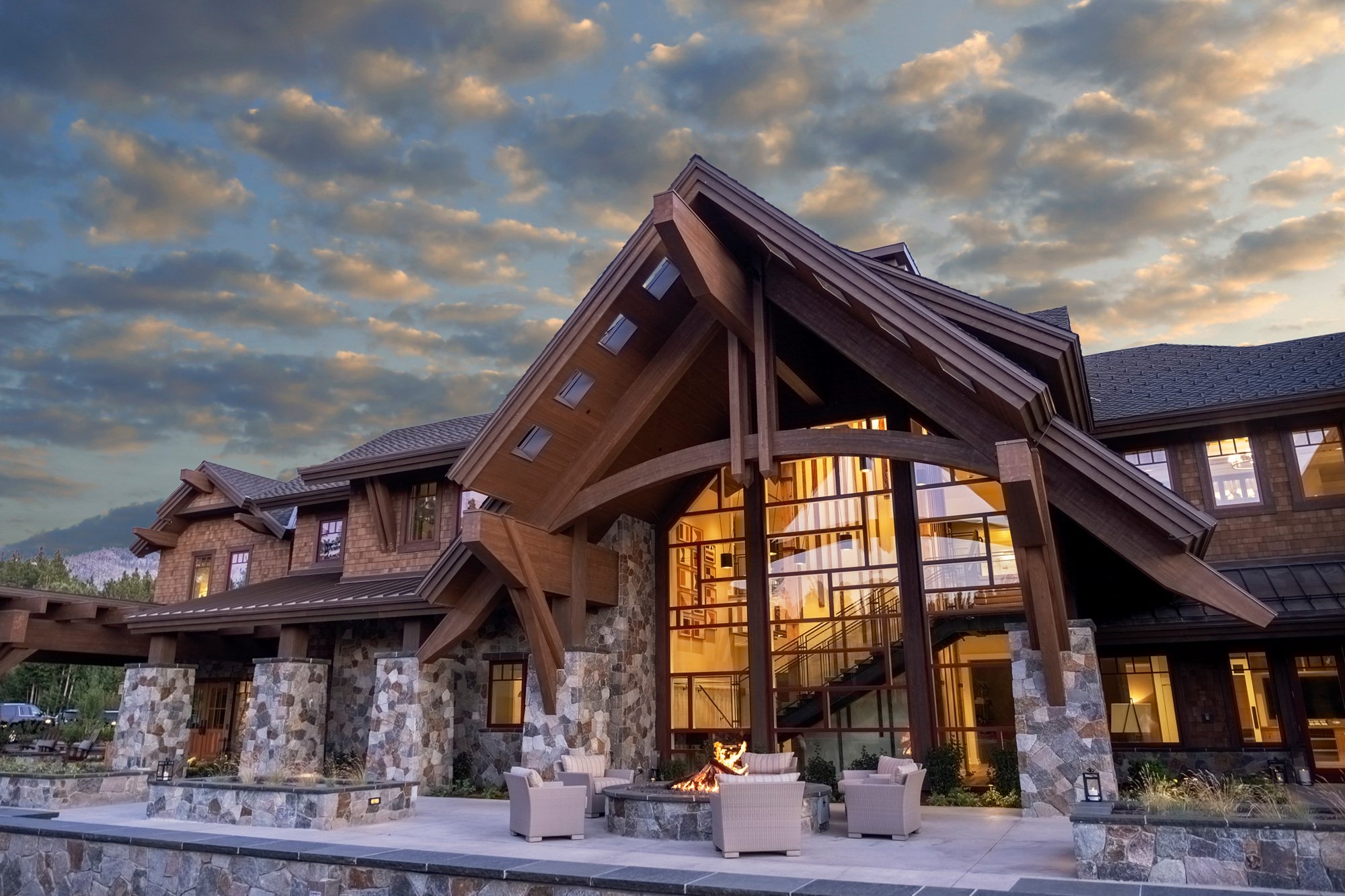This image captures a rustic mansion reminiscent of a lodge, basking in the warm glow of evening light under a blue, yet increasingly cloudy sky. The structure is primarily built with cedar siding and stone, featuring prominently wooden beams and rock-wrapped pillars. The mansion's two floors exhibit a harmonious blend of natural materials; the first level is constructed with various shades of stone—light gray, gray, light brown, and brown—while the second level is adorned with brown wooden siding. The roof, partially visible from the ground-level perspective, appears to be made of black or brown tiles.

Centrally framed in the photograph is a welcoming archway leading into the mansion, complemented by a stone fireplace with a live fire, surrounded by five beige chairs arranged around it. This inviting feature rests on a platform near the entrance. Through the archway, the interior of the mansion glows warmly, revealing stairs that lead to the upper floor, indicating the building's multi-level nature. Additionally, lights hang like lanterns, enhancing the rustic aesthetic. Off to the left side, partially visible, is a parking lot and surrounding greenery, with distant mountains adding to the scenic background.